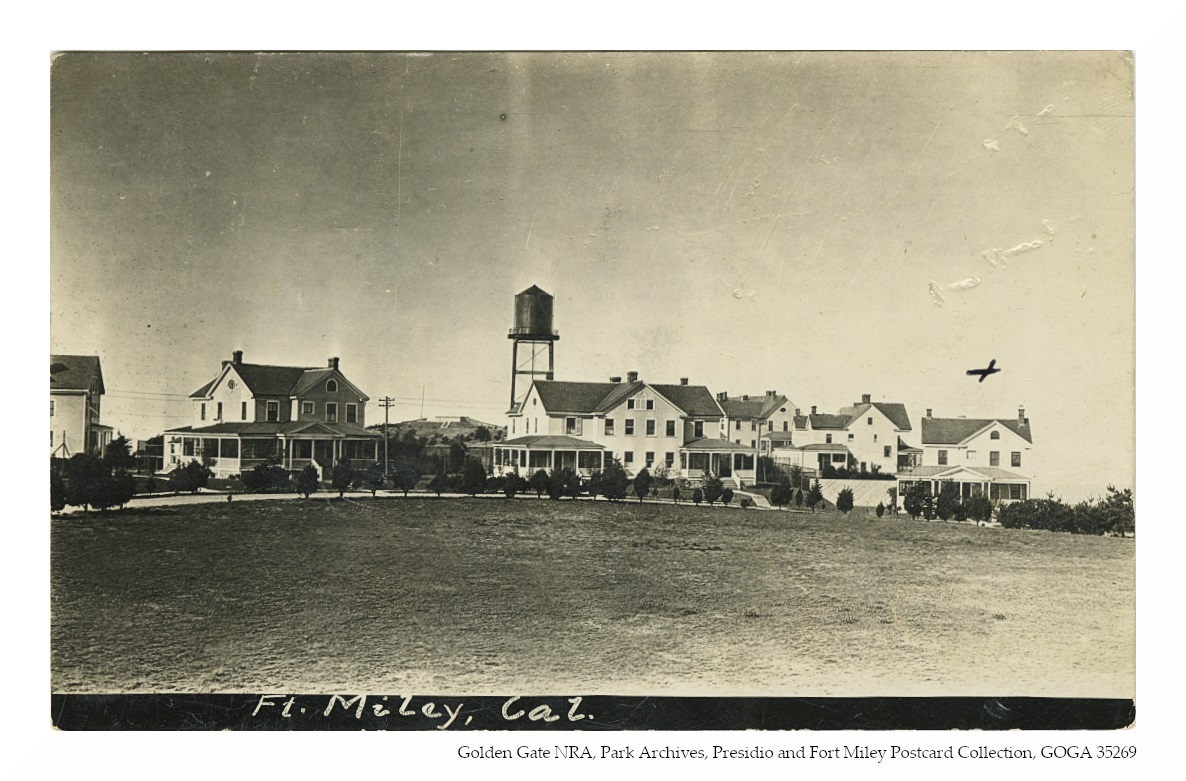This black and white photograph, part of the Golden Gate NRA Park Archives Presidio and Fort Miley Collection, depicts a historic scene from Fort Miley, California. The faded image, which has an old, yellowed tint, features a collection of five or six two-story homes overlooking a hill. The photograph is taken from an elevated vantage point, revealing a small airplane flying above the houses. In the background, a prominent water tower stands tall. The foreground of the image shows a field bordered by a sidewalk lined with short trees and bushes, with telephone lines visible, adding to the sense of bygone times.